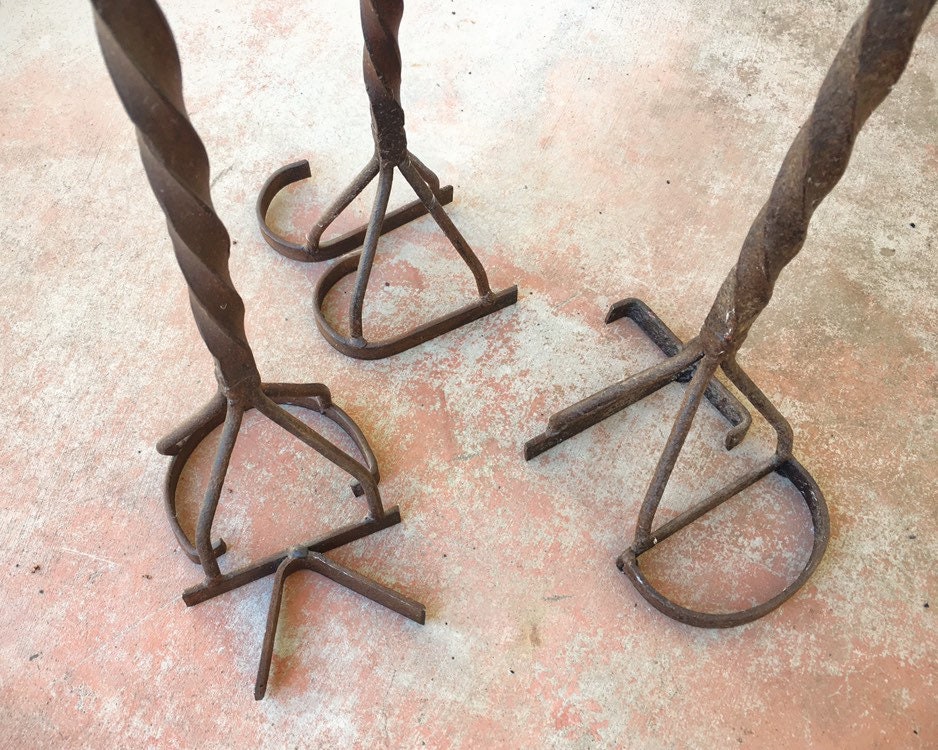This image showcases three branding irons used by cattle ranchers, each intricately designed with iron letters to mark cattle with ownership. The branding irons are arranged to form an equilateral triangle, with each iron resting on its letters that serve as the base. The iron at the top point of the triangle is marked "JJ," the one at the right point is "TD," and the one at the left is "CK." The letters are slightly tilted, all pointing in the same direction, roughly around one or two o'clock. The irons display a mix of rusted red and black, indicating some weathering.

The setting is a concrete floor that was once painted red, evident from the flaked remnants of red paint revealing the white concrete beneath. Despite the aged and worn look of the floor, it appears sturdy. This photograph might have been taken inside a workshop or storage area, where equipment is kept and maintained. The overall scene evokes a sense of rustic utility, grounded in the practice and tradition of cattle ranching.